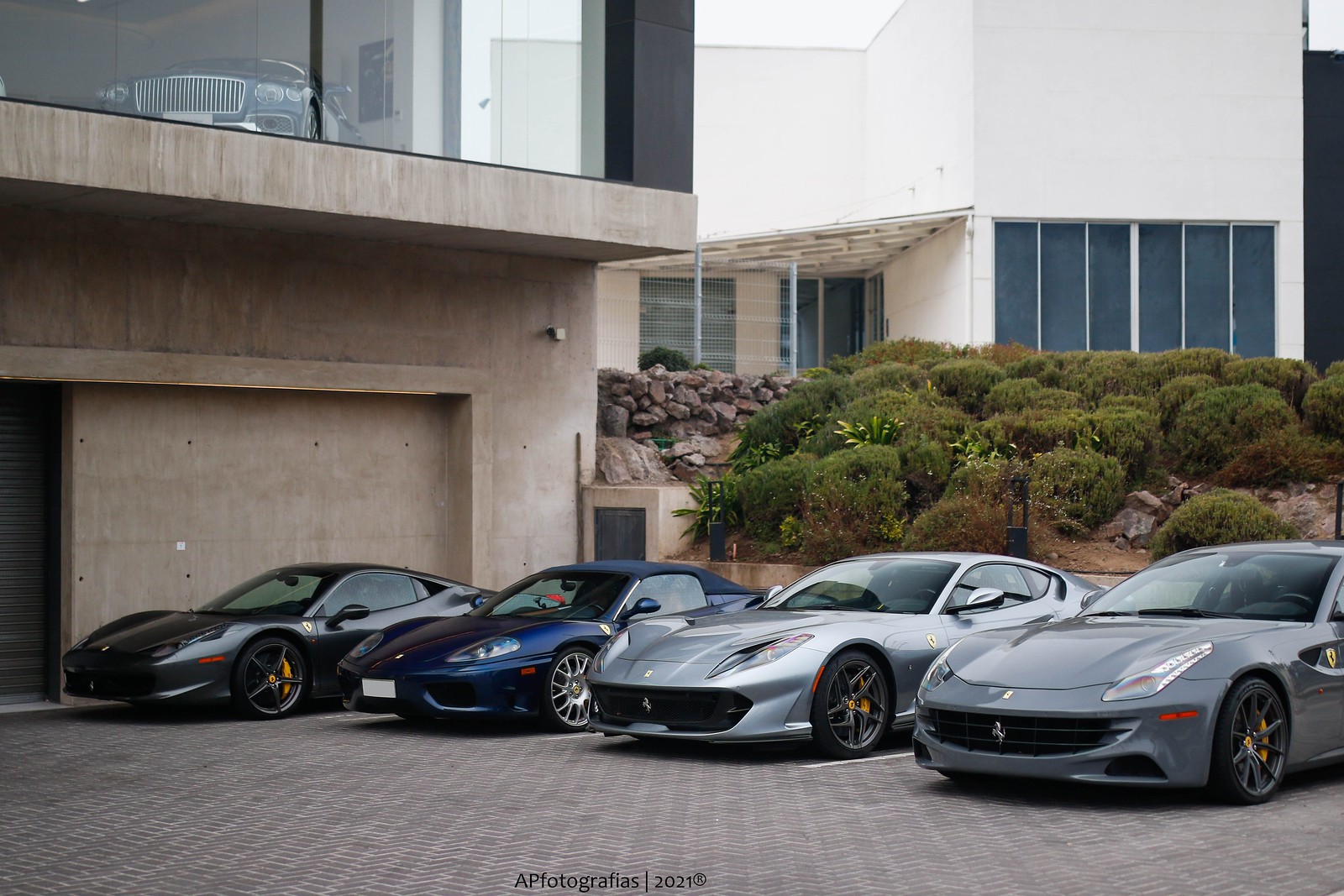The photograph, taken in 2021 and recognizable by an "R" symbol, depicts an outdoor scene featuring four pristine sports cars lined up meticulously on a brick-laid driveway. These high-performance vehicles include one black car, one dark blue, and two metallic silver, each gleaming with a well-maintained shine. The backdrop showcases a modern building with a unique architectural design, blending white and gray hues with a tan or brown brick wall. The second story of the building, resembling a showroom, reveals the front grill of another car through large black-framed windows. Below this, green shrubs and decorative rocks add a touch of landscape beauty beside the stone ledge of the building.